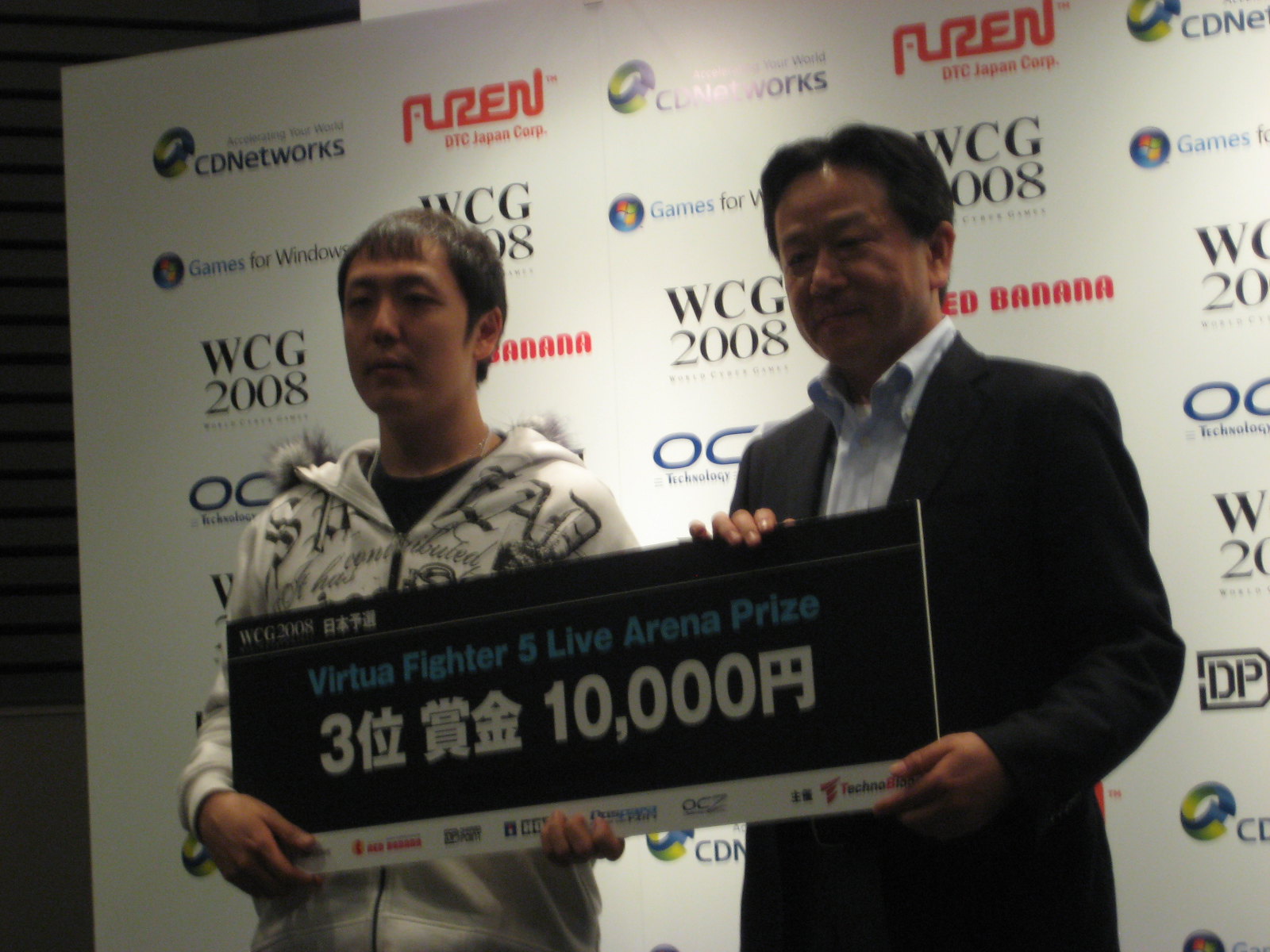This photograph captures a celebratory moment featuring two Asian men on stage, proudly holding a placard that reads "Virtua Fighter 5 Live Arena Prize 3," followed by Chinese characters and the figure "$10,000." The man on the left, presumed to be the fighter, sports short black hair and a white hoodie adorned with black script, gripping the bottom of the sign with both hands. The man on the right, likely the promoter or manager, has slightly longer black hair and is dressed in a black blazer over a blue collared button-down shirt, holding the sign with one hand on the bottom and the other on top. Positioned against a backdrop, the slightly side-angled and low-resolution photo features a large white wall poster filled with a myriad of sponsor logos, including the prominent "WCG 2008" and "Games for Windows." The colorful logos contrast against the white background, highlighting the event's esteemed sponsors.